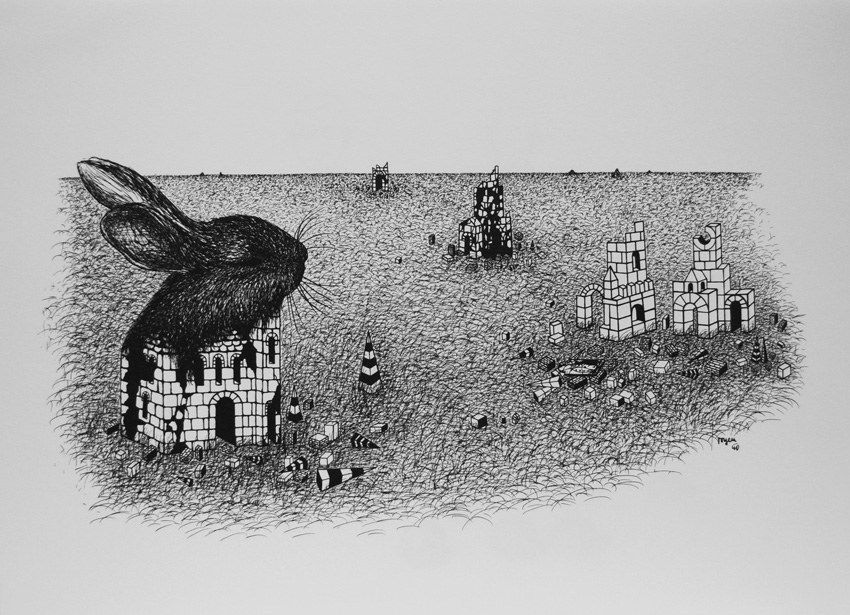The hand-drawn black and white image, set against a light gray background, features a surreal landscape dominated by a peculiar architectural scene. On the left side of the drawing, there is a detailed stone building with a square-brick construction and an arc-shaped entrance at the front. Atop this building, a strikingly large head of a black rabbit with very long ears is prominently displayed, its eyes closed in a serene expression. Surrounding this structure, in the foreground, are scattered traffic cones with black and white horizontal stripes, some of them standing upright while others are toppled over.

To the right of this primary building, there are two additional white buildings, also built from square bricks and featuring their own entrances. These buildings appear slightly disordered, resembling discarded or old castles. The composition extends across the entire image, with no single centralized focus, creating a sense of intriguing complexity. The overall impression is one of a unique and intriguing piece of artwork, likely part of an artist's personal collection, rendered meticulously in shades of black, white, and gray.